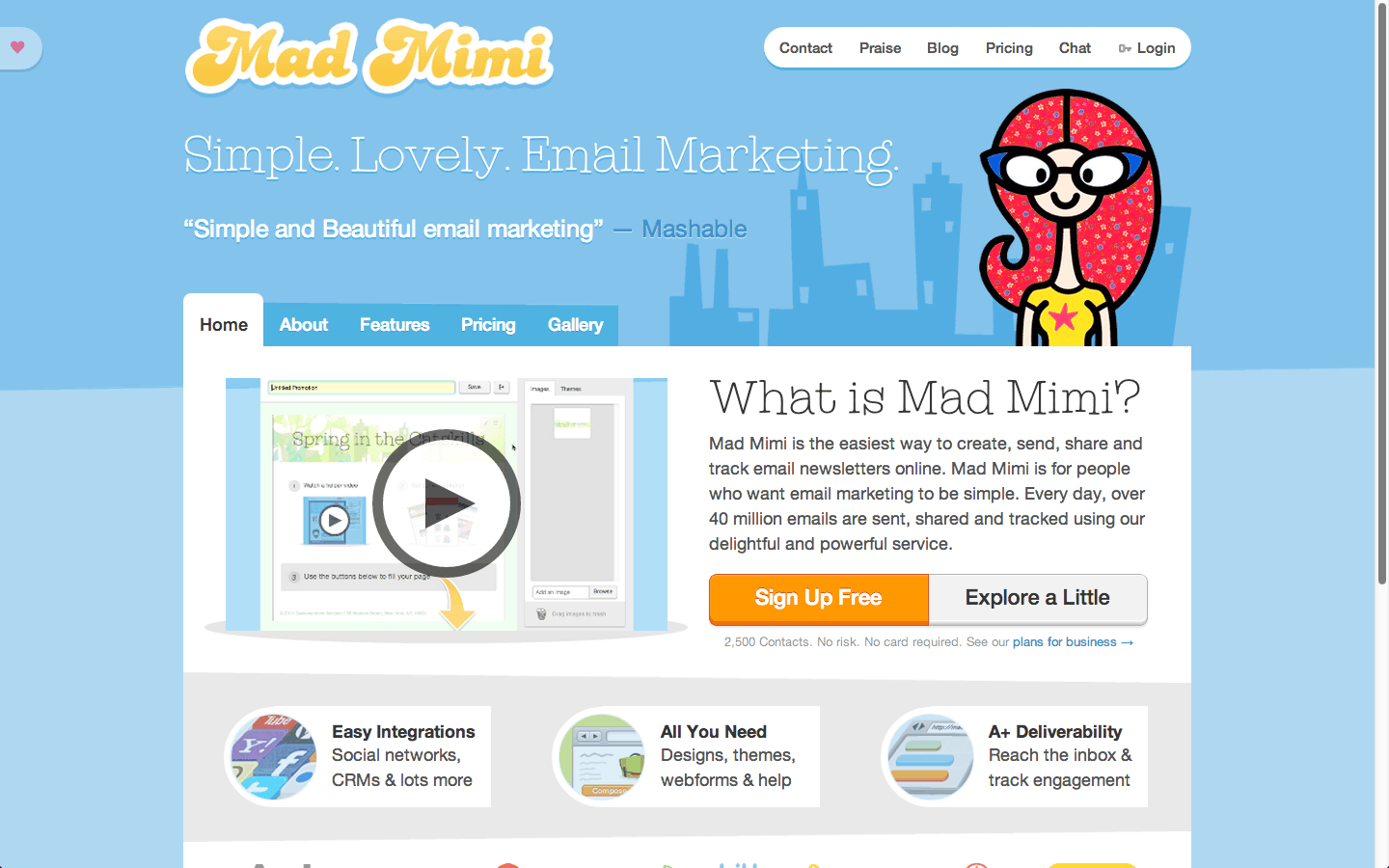The image features a vibrant blue background adorned with a cityscape silhouette of tall blue buildings. At the top, in bold, bubble-style yellow text, it prominently reads "Mad Mimi." Just below, in a similar fashion, it states "Simple Lovely Email Marketing." To the right, there is a cartoon character with distinct features: large, oversized blue-rimmed glasses, red curly hair, and a yellow shirt emblazoned with a red star.

To the left of the character, the phrase "Simple and Beautiful Email Marketing – Mashable" is displayed. Beneath this, the word "Home" is written in black next to a black play arrow, indicating a video can be played. Adjacent to this, text reads "What is Mad Mimi?" followed by an explanation that "Mad Mimi is the easiest way to create, send, share, and track email newsletters online. It's designed for people who want email marketing to be simple."

At the bottom, there are three distinct call-to-action options: 
1. A red/orange square inviting users to "Sign Up Free."
2. A gray square offering to "Explore a Little."
3. Three white squares at the very bottom providing further options: "Easy Integrations," "All You Need," and "A Plus Delivery," which claims "Reach the Inbox and Track Engagement."

Each element within the image is carefully crafted to convey the simplicity and effectiveness of Mad Mimi's email marketing solutions.